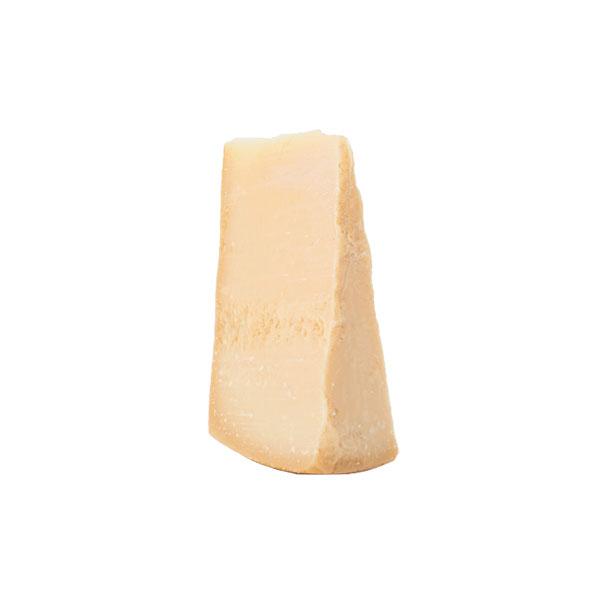In the center of an all-white background, there is an upright wedge of cheese. This wedge stands on its wide, curved base, exhibiting a light, off-white color that sits between yellow and white. The cheese appears clean and well-defined, with brown edges, especially noticeable along the curved bottom where it has likely been cut from a cheese wheel. The surface looks slightly crumbly, suggesting it might be a softer variety of cheese.